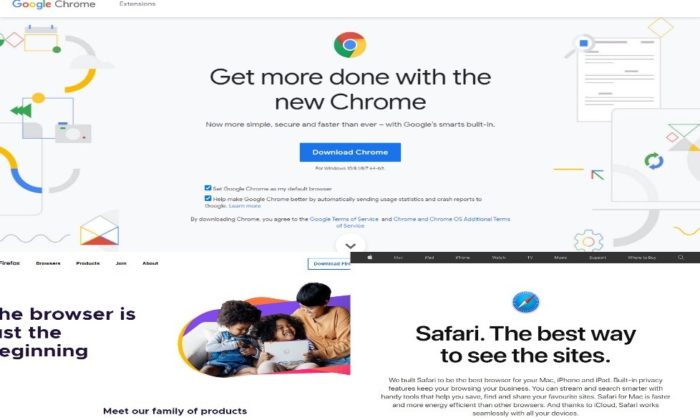The image showcases a composite web browser start page, prominently featuring the Google Chrome homepage in the center. The upper left-hand corner displays the Google Chrome logo alongside an extensions option. The central portion of this page highlights a large Google Chrome icon with a promotional message: "We're done with the new Chrome. Now much more simple, secure, and faster than ever with Google Smart built-in." Below this message is a blue "Download Chrome" bar. 

In the lower portion of the page, there are several check marks, likely representing license agreements, although these are difficult to read due to resolution limitations. Beneath the primary Google Chrome section are smaller segments representing the start pages of other web browsers. On the left is Firefox, with its smaller interface. On the right is Safari, featuring its icon and a tagline, "The best way to see the sites," accompanied by various menu options.

The image illustrates the competitive landscape of web browsers, with Google Chrome noted as the most widely used, Safari as Apple's offering, and Firefox as the underutilized but still supported alternative. However, text clarity is compromised due to low resolution, making some details hard to decipher.